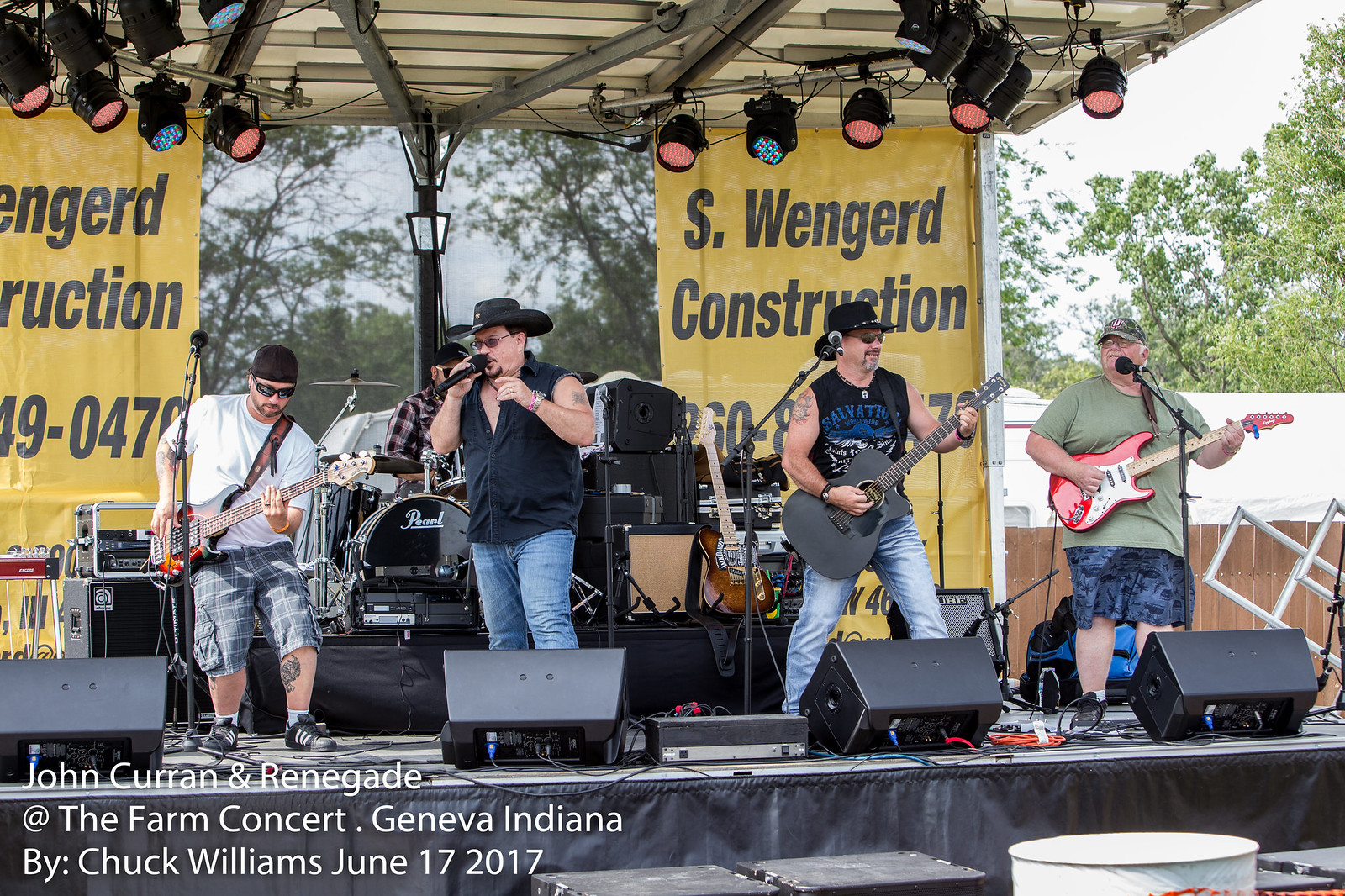The image captures an outdoor rock concert featuring the band John Curran and Renegade at the Farm Concert in Geneva, Indiana, on June 17, 2017. The stage, covered and adorned with blue and red lighting, is backed by a large yellow banner reading "S. Wengerd Construction" in black letters. The band comprises five members: 

Starting from the left, a man plays the bass guitar, dressed in a black hat, white t-shirt, gray cargo shorts, and black shoes. Next to him, the lead singer has a black cowboy hat, black vest, and blue jeans, passionately holding a microphone. To the singer's right, another musician strums a black acoustic guitar, wearing a black tank top, black cowboy hat, and lighter blue jeans. Further right, a larger guitarist plays a striking red and white electric guitar, clad in a green t-shirt, green ball cap, blue shorts, and black sneakers. Positioned behind the lead singer, the drummer sports a checked shirt, surrounded by his drumming equipment.

The lower-left corner of the image features white text that reads, "John Curran and Renegade at the Farm Concert, Geneva, Indiana, by Chuck Williams, June 17, 2017." In the backdrop, green trees are visible, enhancing the outdoor ambiance of the lively concert. The stage setup includes black curtains and four speakers in front of it. Flanking the stage are two yellow banners with black text and additional numbers beneath the construction company's name. In front of each band member, there are monitors, barrels, and some kind of square boxes on the stage floor.